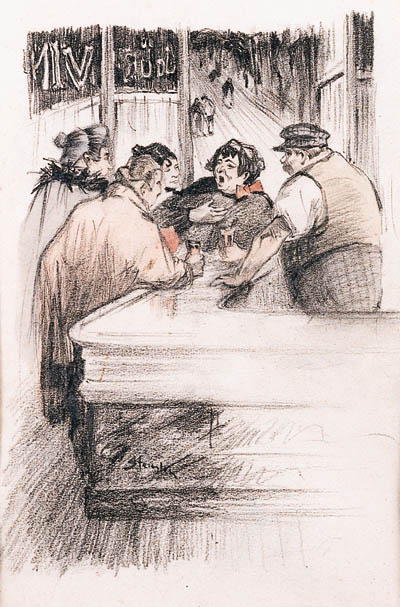The image is a heavily sketched, predominantly black and white drawing of a bar scene with minimal use of colors like tan, gray, and hints of red. In the foreground, there is a stark white bar with black sketchy edges extending from the right side and turning towards the back of the image. Behind the bar, a large, round man, who is white and wearing a checkered cap, tan vest, white shirt, and dark striped pants, leans over the bar towards a group of four women. These women, who appear to be elderly and are dressed in heavy coats, are engaged in an intense conversation. The woman on the far right wears a black coat adorned with a purple and pink bow, and she, along with the woman to her left in a tan coat, holds a cup of amber liquid. The scene includes a lot of dynamic pencil shading, adding depth to the black and white aesthetic. In the background, an open door reveals a street with basic pencil-drawn figures, enhancing the scene's bustling atmosphere.